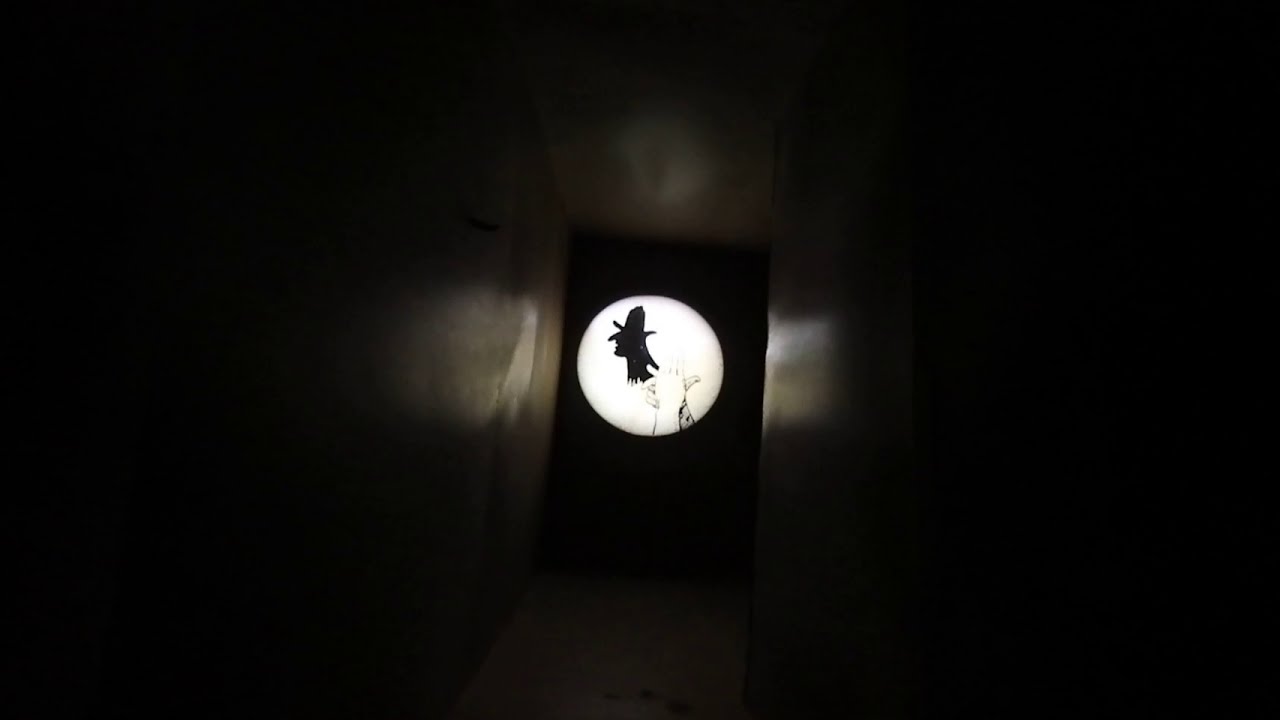The photograph showcases a predominantly dark, narrow hallway with black walls that extend unevenly, the left wall being longer than the right. At the end of the hallway, there is a projection displayed on the black wall. The focal point of this projection is a glowing red circle that prominently features a sketched image of a witch's head, complete with a pointy nose and witch hat. Directly below and to the right of the witch's head, the red circle also illuminates a sketch of two hands clasped together, forming the shape of the witch's face and hat through shadows. The light from the projection subtly illuminates portions of the walls and ceiling, which are a dark beige or brown color. The setting is so dimly lit that the primary sources of light are the projected red circle and its faint reflections on the surrounding walls. The entire scene conveys a mysterious and eerie atmosphere, accentuated by the monochromatic palette and the haunting imagery of the witch.